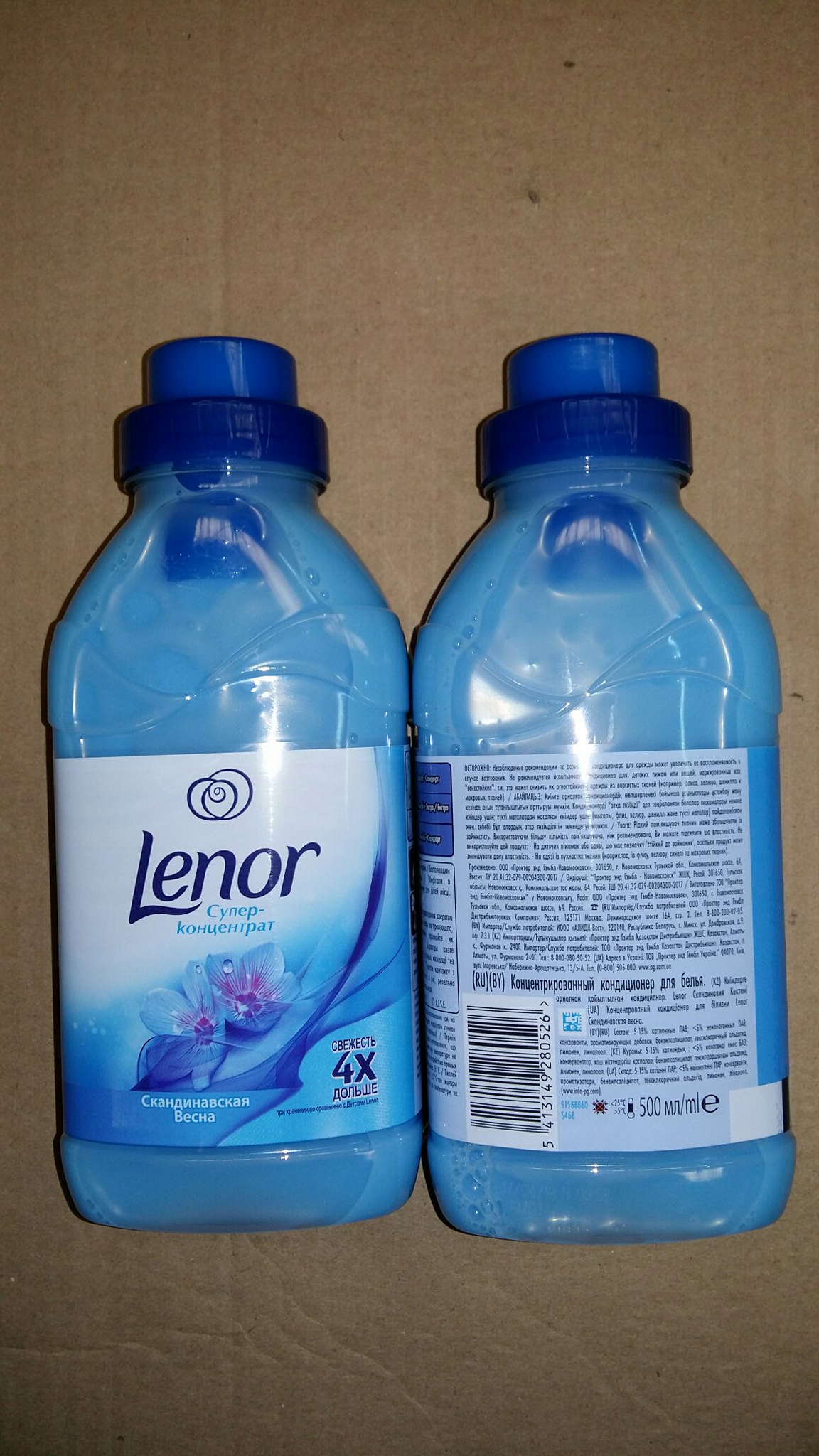A detailed photograph features two identical bottles of Lenor laundry detergent, placed on a brown cardboard surface. The bottles are a vibrant blue with darker blue caps, and both appear to be full. One bottle is positioned upright, showcasing the front label, while the other is lying down, displaying the back label. 

The front label of the upright bottle prominently displays the brand name "Lenor" in large white text, accompanied by a second line of text in Cyrillic script, suggesting it is a Russian product. Ornate illustrations of blue and purplish jasmine flowers embellish the bottom of the label. A notable text at the lower part of the label states "4X," indicating the product's enhanced strength or longevity.

The back label of the bottle lying down reveals a wealth of information, including usage instructions, ingredient details, and a barcode for scanning. This information highlights the product’s commitment to transparency. The overall presentation and vibrant colors of the bottles give them a fresh and appealing look.